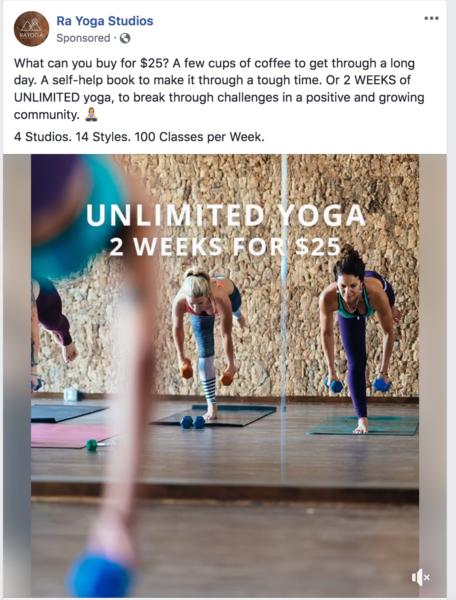**Detailed Caption:**

In this vibrant, portrait-oriented screenshot captured from a mobile device, we see a social media post, most likely from Facebook, though distinct platform identifiers are missing. At the top of the post, the name "Raw Yoga Studios" is prominently displayed in an unusual blue font. To its left, there is a unique logo comprising the words "Right Yoga" with two pyramid-like designs above it set against a brown background. 

The post reads, "What can you buy for $25? A few cups of coffee to get through a long day, a self-help book to make it through a tough time, or **two weeks (in all caps) of UNLIMITED (all caps) YOGA** to break through challenges in a positive and growing community. Four studios, 14 styles, 100 classes per week. **Unlimited Yoga: Two Weeks for $25.**

The bulk of the screenshot is dominated by an engaging image of three women poised in front of a mirror, reflecting their dedication. They are balancing on one leg while holding weights, embodying strength and focus, the essence of the yoga journey promoted by the studio. This visually compelling photograph encapsulates the supportive and dynamic environment that Raw Yoga Studios aims to foster.